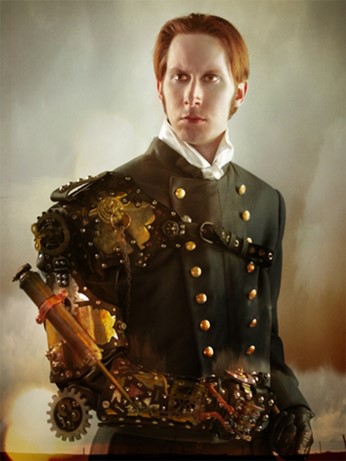This photograph features a serious-looking gentleman with short reddish hair, dressed in a striking steampunk-inspired outfit. He is shown from the waist up, with a light brown background that complements his attire. His left hand is adorned with a black leather glove, and his right arm is an intricate mechanical marvel, complete with brass gears, rivets, screws, a hydraulic piston, and a syringe-like device, invoking a parallel to Edward Elric's automail arm from "Full Metal Alchemist." 

He wears a double-breasted coat with white collar and brass buttons, styled in an old Victorian naval fashion. The coat, primarily black, is detailed with steampunk motifs including metal shoulder straps, leather belts, small spikes, and decorative gears, adding an air of both sophistication and industrial flair to his ensemble. The man's expression is grim and focused, his clean-shaven face contributing to his stern appearance. Behind him, a light brown backdrop provides a subtle contrast to his dark, elaborate outfit.